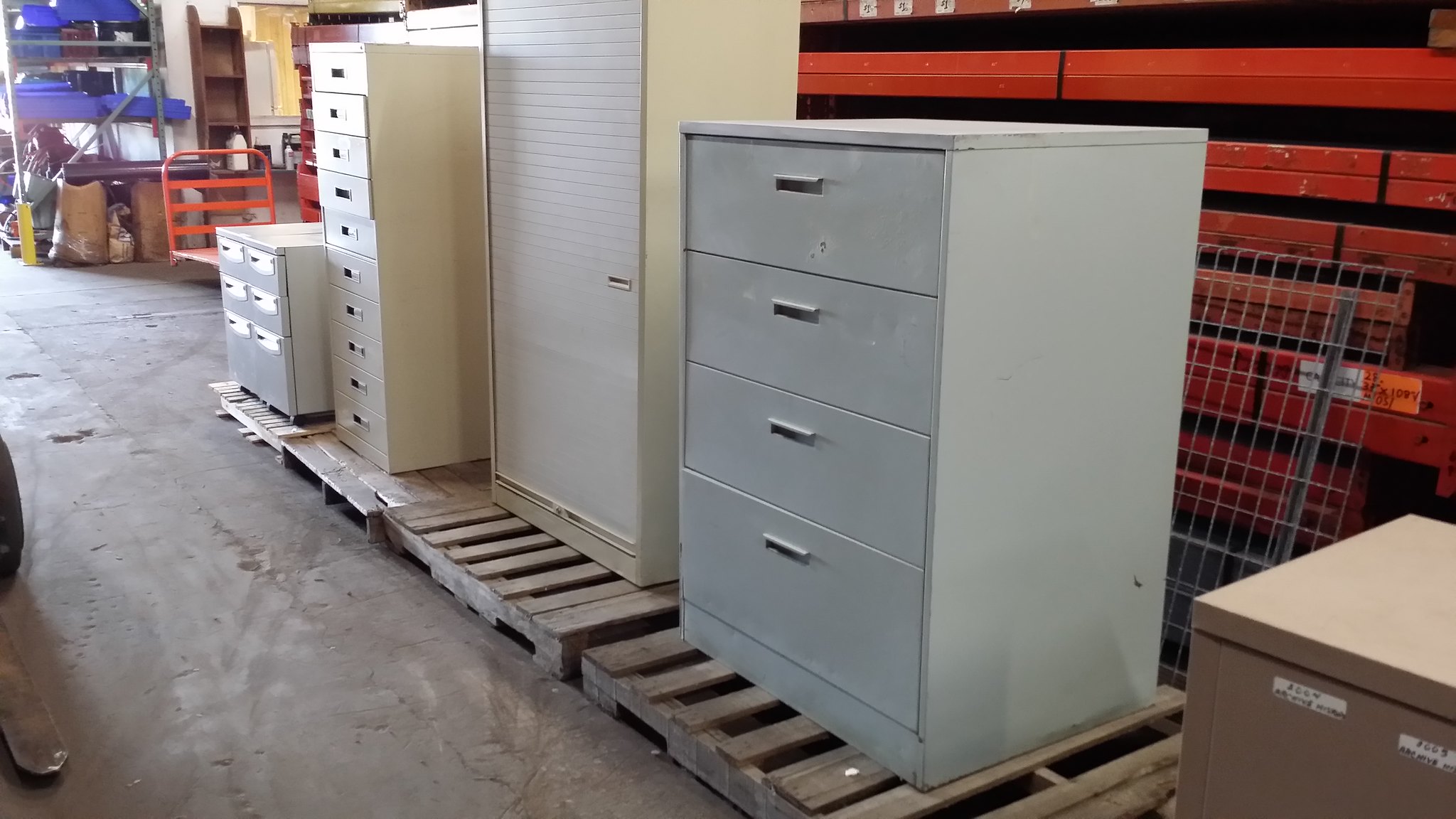The photograph depicts a typical warehouse scene with a row of various filing cabinets placed atop wooden pallets on a concrete floor. The cabinets, each differing in size and shape, include a tall grey one with four long drawers, a light grey cabinet with a door resembling a wardrobe or closet, a cream-colored one with several small drawers similar to an index card filing system about six feet tall, and a smaller cream-colored chest of drawers. Arranged at a 45-degree angle from the left, the cabinets are positioned in front of some red shelving units visible in the background. The warehouse has white walls, and the floor appears somewhat unclean. Additional features include blue and metal shelves in the distance, some brown items underneath the shelves, a forklift's tongue on the left edge of the photo, and a corner with dollies.